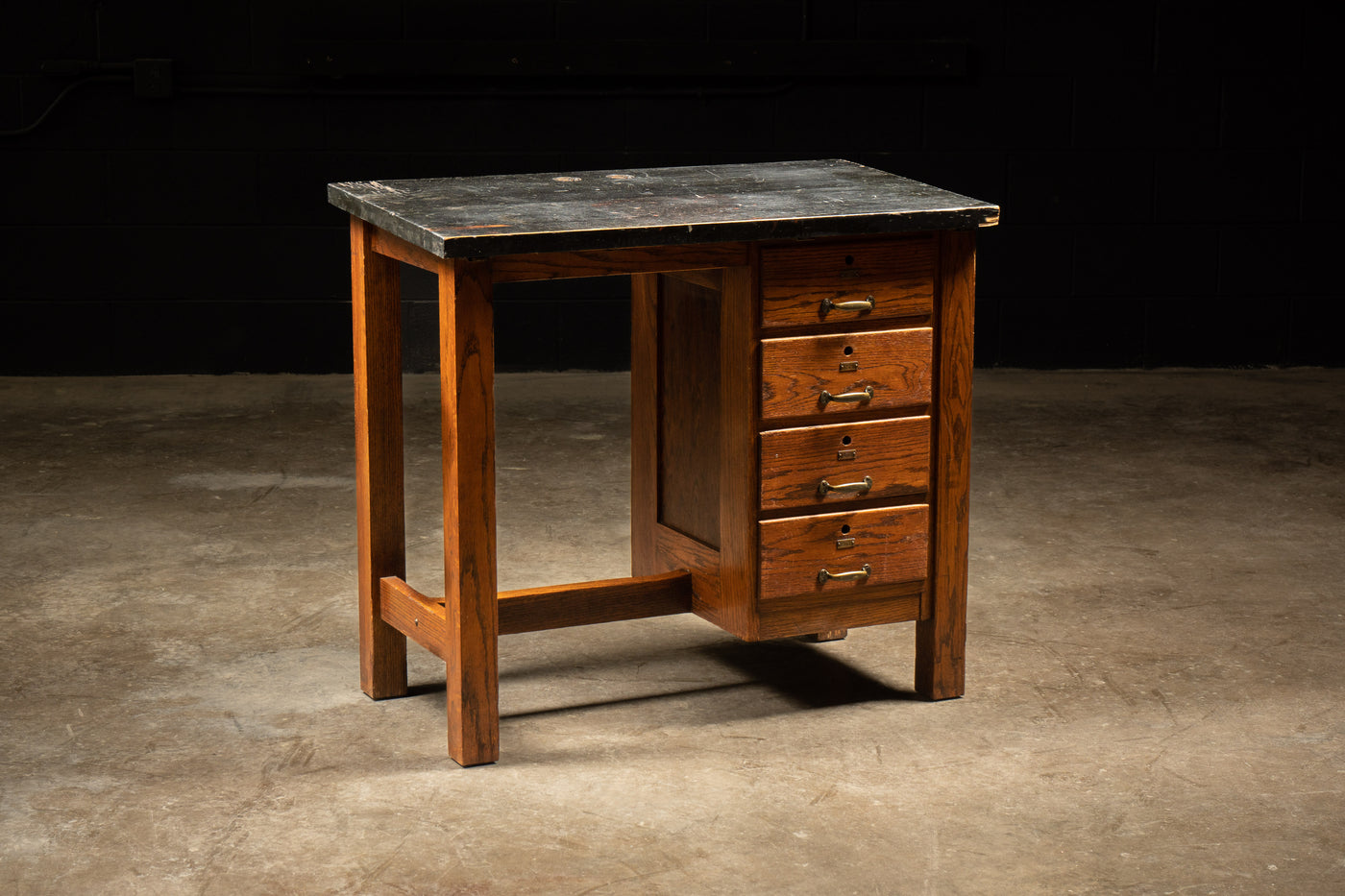This image captures a centrally positioned wooden desk with a refinished black top, standing alone in a room. The desk exhibits a dark wood tone and features four closed drawers on the right, each equipped with a keyhole and golden or brass handles. The desk has four cuboidal legs and a connecting support bar on the left-hand side. The background's upper half is black, while the lower half is tan or brown, resembling a cement floor with a tannish gray hue. The scene is devoid of people, text, or other imagery, emphasizing the desk against the flat, monochromatic backdrop.